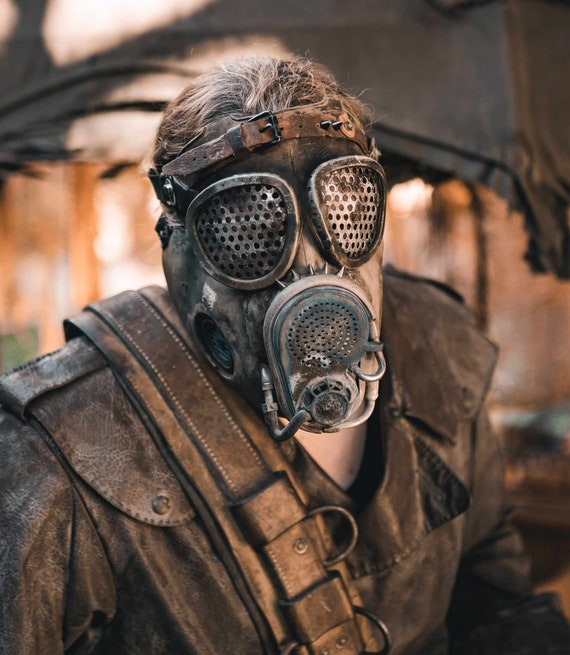This color photograph captures a close-up shot of an individual from mid-chest up, seemingly prepared for a harsh, possibly apocalyptic environment. The person, who appears to be a man, has fair skin and messy light brown hair. They are donning a worn, slightly dirty, brown leather jacket paired with a cross-body leather utility belt strapped over their right shoulder, designed with metal links for attaching tools.

Covering the person's face is an imposing, weathered gas mask with a distinctly steampunk aesthetic. This full-face mask features mesh screens over the eyes that resemble bug eyes, small black holes, and metallic spikes on the rebreather portion. A prominent leather strap with a belt buckle runs across the forehead of the mask. 

The background is blurred but indicates the presence of a dark brown tent or structure and suggests outdoor, daytime lighting with shadows cast by natural light. This meticulously detailed outfit and the beaten-up mask hint at a scenario torn from an apocalyptic or dystopian scene, as if from a movie still.